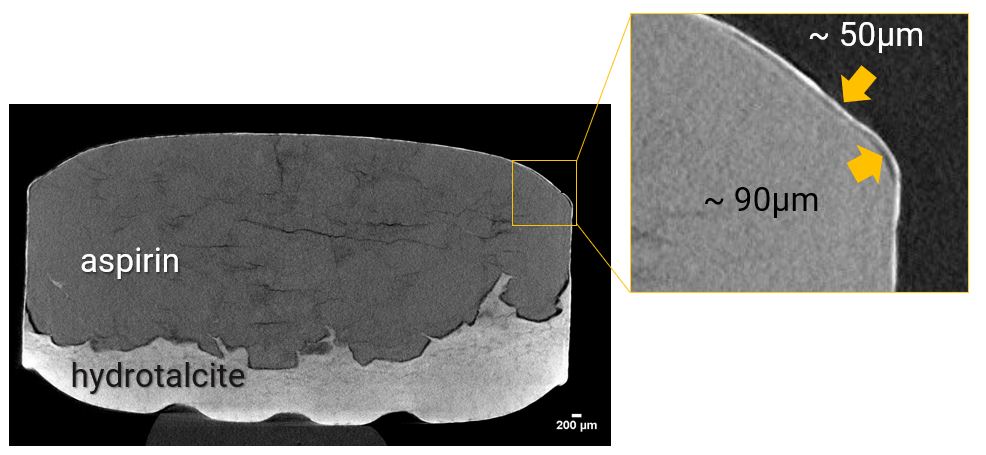The image features two diagrams set against a black background, illustrating the composition of a substance, specifically a medication. The larger diagram on the left showcases an oblong shape with rough edges, divided into two distinct layers. The upper gray layer is labeled "aspirin" in white text, while the lower white, zigzag-edged layer is labeled "hydrotalcite" in black text. At the bottom right corner of this diagram, "200 μm" is noted in small white text. Highlighted in the upper portion of this image is a yellow-bordered square. The diagram on the right offers a magnified view of this yellow square, detailing the two layers further. In the gray area, corresponding to the "aspirin" layer, a wavy line indicates a thickness of approximately 90 μm. Two yellow arrows point towards the surface, one from the gray area and another from the black surrounding area, with the latter indicating a measurement of approximately 50 μm. This comprehensive depiction suggests an analysis of the tablet's microstructure, with clear text annotations and precise layer distinctions.